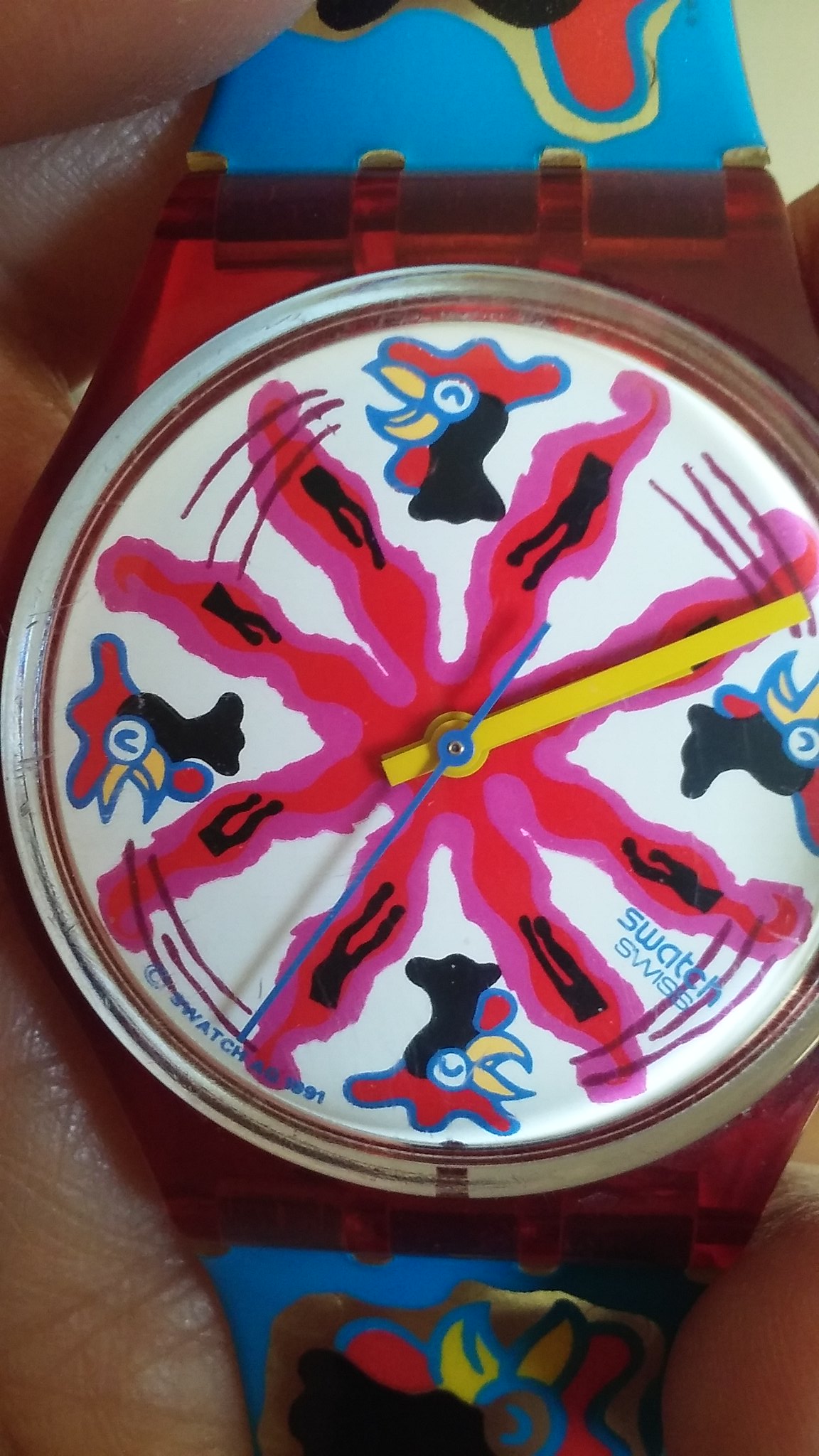This color photograph showcases a close-up of a novelty watch held by a person with dark brown skin, visible in the background towards the upper and lower left corners. The watch has a round face adorned with cartoon depictions of roosters located at the 3, 6, 9, and 12 positions, while in between these positions, large crooked lines with red and pink outlines and black splotches can be seen. The watch features two overlapping yellow hands, a smaller blue second hand, and lacks numeric indicators, making it difficult to discern the exact time. It is encased in a silver frame and is attached to a blue strap embellished with intricate orange, green, and brown designs. The upper right-hand corner of the image shows a greyish-green background, adding contrast to the vibrant colors of the watch.